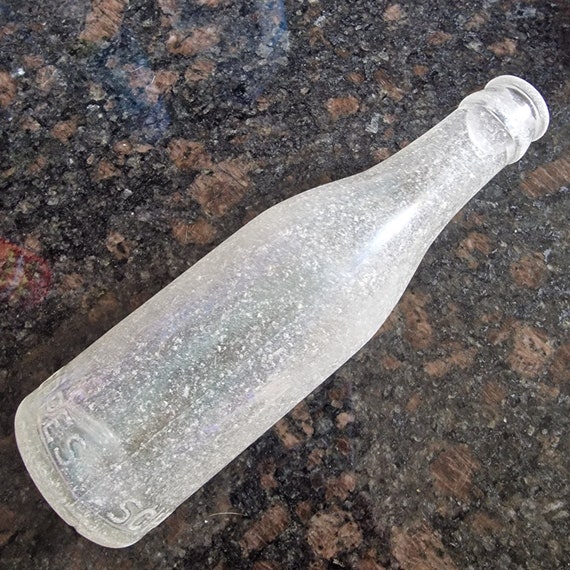The image is a detailed color photograph, most likely taken indoors, of a weathered glass bottle lying diagonally on a countertop. The countertop appears to be a black and brown-orange mottled stone, possibly marble, with a glossy finish in some areas, particularly the upper left corner, and a duller look on the lower sections. The glass bottle, positioned with its base on the lower left and its top towards the upper right, has a cylindrical shape that narrows towards the top, resembling an old style bottle. Its cap is missing, and the glass itself is heavily aged and white, covered in white specks and calcification, suggesting it may have been buried or exposed to the elements for a long time. The base of the bottle features raised lettering, partially visible, with "EPPES" on the left and "SCH" on the right, indicating it is likely a Schweppes bottle. The bottle's condition and positioning against the distinct countertop add layers of texture and history to the photograph.